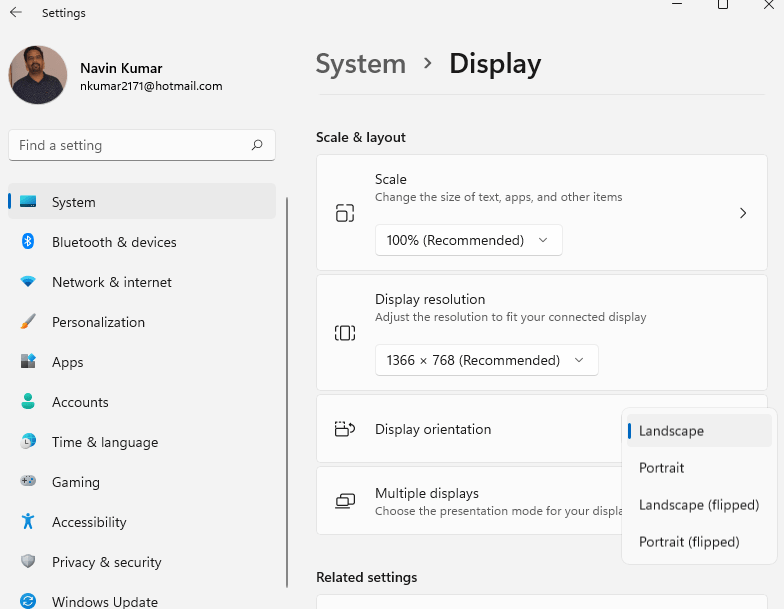In this detailed image of a Windows settings menu, the primary focus is on the "System" settings. At the top left corner, the word "Settings" is displayed with a left-pointing arrow next to it. Directly beneath this, a profile picture of a man is visible, alongside which the name "Navin Kumar" and his email address "nkumar217@hotmail.com" are displayed. 

On the right side of this profile information, the word "System" is highlighted, with an additional indication pointing towards "Display," which is colored in black. 

To the left side of the image, there is a search bar labeled "Find a setting." Below this search bar, a list of different categories is organized sequentially. The categories listed are: System, Bluetooth and devices, Network and internet, Personalization, Apps, Accounts, Time and language, Gaming, Accessibility, Privacy and security, and lastly, Windows Update at the very bottom.

Towards the top-middle section of the image, the label "System - Display" is displayed again. Underneath this header, the "Scale and Layout" section is revealed, which contains several configurable options. The first box allows users to change the scale, adjusting the size of text, apps, and other items. The second box pertains to the display resolution, providing the functionality to adjust the resolution for a connected display. The third box offers settings for display orientation, and the fourth box manages multiple displays.